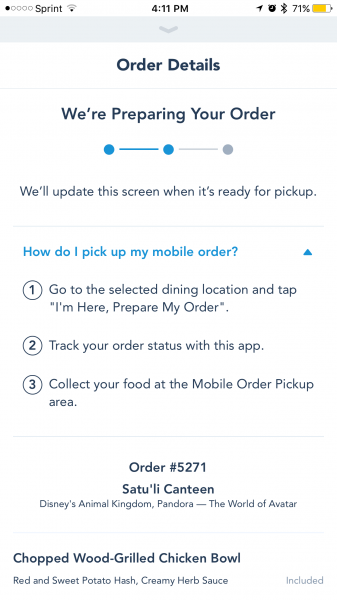The image depicts an online order details screen on a smartphone. In the top left corner, the phone is connected to Sprint, but the signal strength is weak with only one out of five circles filled in and a single bar of Wi-Fi signal. It is 4:11 p.m., and location services, alarm, and Bluetooth are all activated. The battery is at 71% and appears yellow.

A drop-down menu reveals "Order Details" where the status is "We're preparing your order." Below this, a visual timeline marked by three circles and connecting lines is shown—two circles are filled, indicating progress. The message below reads, "We'll update the screen when it's ready for pickup."

Further instructions in aqua blue text and a triangle pointing up are provided: "How do I pick up my mobile order?" Steps are listed as follows:

1. Go to the selected dining location and tap 'I'm here, prepare my order.'
2. Track your order status within the app.
3. Collect your food at the mobile order pickup area.

The order number is 5271, placed at Disney's Animal Kingdom, Pandora – The World of Avatar. The order consists of a chopped wood-grilled chicken bowl with red and sweet potato hash and creamy herb sauce included.